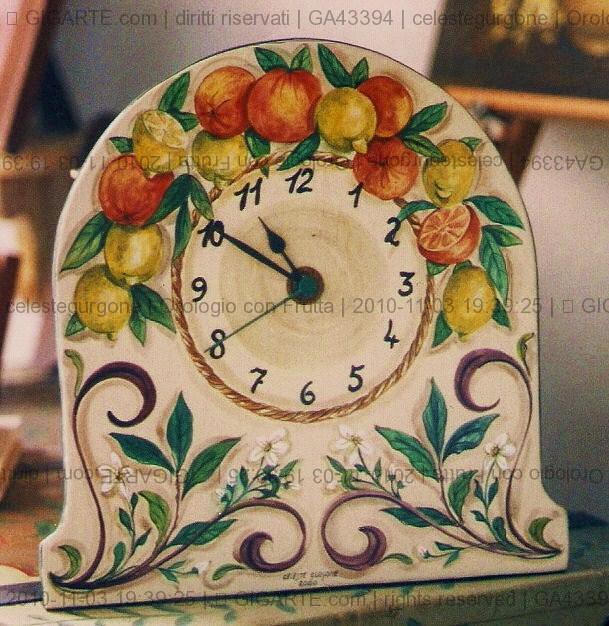This is a color photograph capturing an ornamental clock, likely crafted from porcelain or similar ceramic material. The clock’s design features a rounded top and a square bottom. The clock face exhibits a round white background with black numerals ranging from 1 to 12. The black clock hands are positioned with the hour hand at 11, the minute hand at 10, and the second hand at 8. The upper edge of the clock is adorned with vibrant, detailed illustrations of fruits, including apples, perhaps lemons, and green foliage. Below the clock face, there is an elegant design featuring green leaves and swirling purple patterns. The clock rests on a visible tabletop, set against a plain grey wall. To the left and right of the clock, wooden objects are partially visible. A watermark, consisting of small, dark print with numbers and a partially legible website address, runs horizontally across the photograph at intervals of approximately every two inches.